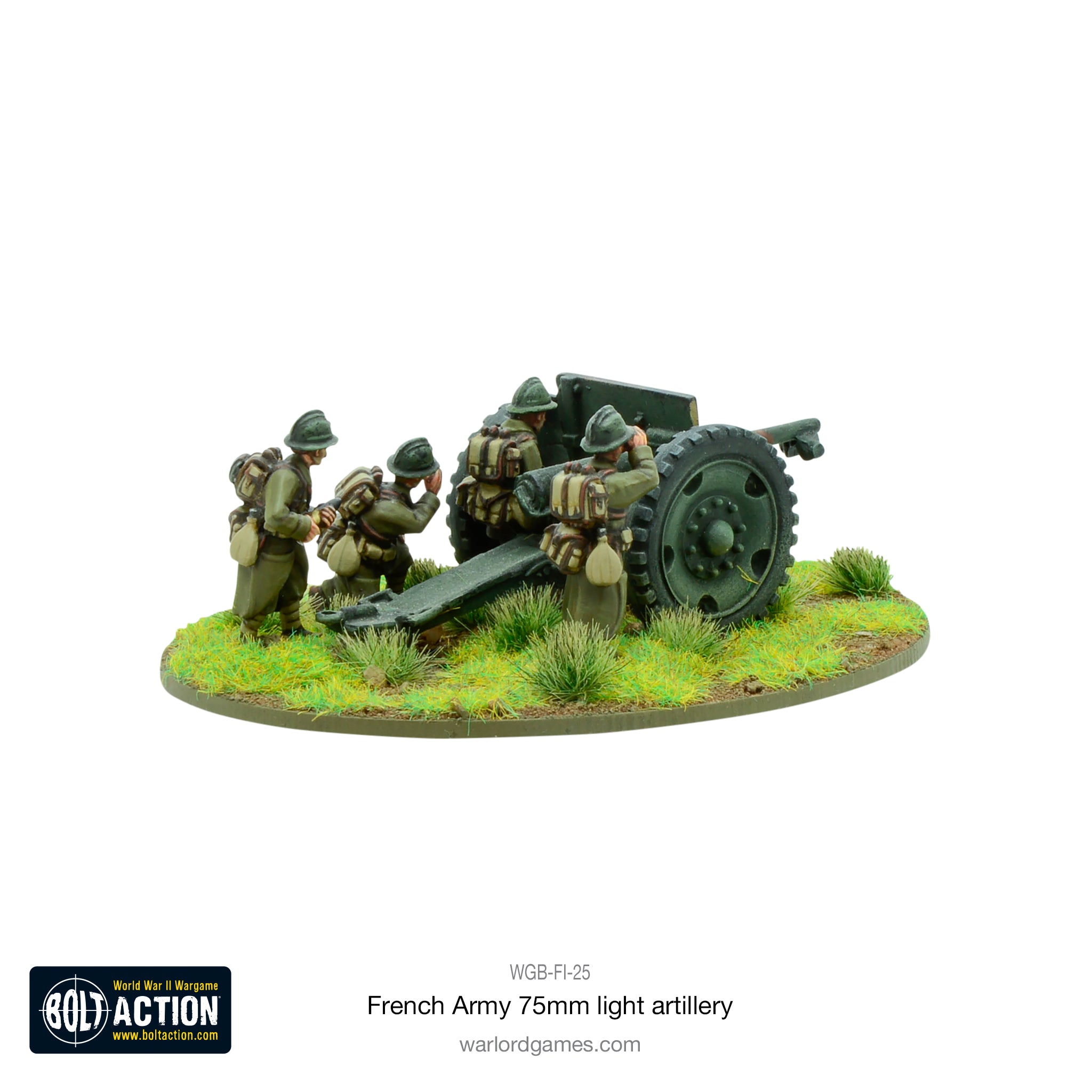The image features a detailed miniature scene depicting a World War I artillery crew in action. The focal point is an artillery gun with large wheels, a metal shield, and a tail-like rod extending to the ground. Four soldiers, dressed in olive green uniforms and dark green helmets, stand behind the gun on a grassy and soil-mottled round platform. Two of the soldiers hold binoculars, scanning the horizon, suggesting they are targeting an enemy. One soldier appears to be firing the gun, while another is hunched over, possibly also using binoculars. The soldiers are equipped with brown and beige backpacks and supplies, including canteens. At the bottom of the image, text reads "Boat Action, World War 2 War Game, www.boataction.com" and "WGB-FI-25, French Army 75mm Light Artillery, www.warlordgames.com," indicating the scale model's product details.